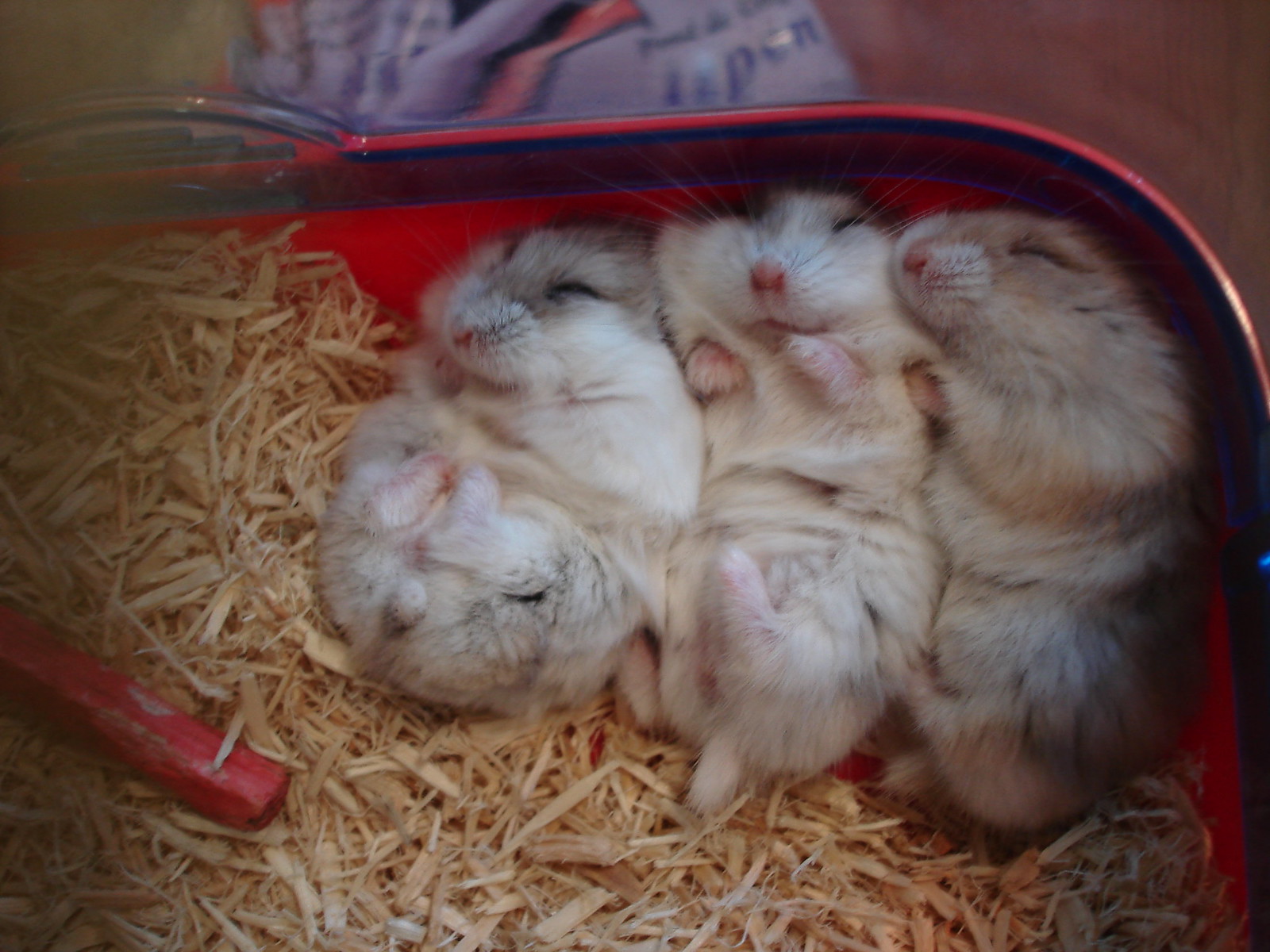This image showcases an up-close view of three baby hamsters, snuggled together in a red, plastic container filled with light-colored wood shavings and mulch pieces. The trio, with their eyes tightly squinted shut like tiny black lines, appear to be in a deep sleep. Their little pink noses and long whiskers are prominently featured. The one on the left, with grayish head fur, has its tiny feet tucked comfortably against its stomach. The middle hamster, a cream-colored one with white patches, shows its tiny pink hands just beneath its mouth, while the hamster on the right, a slightly tan one, lies on its side with one small hand resting against its neighbor. In the background, blurred and faint, are indistinct, possibly elevated objects, suggesting the container rests on a higher surface such as a table. To the lower left, a red handle extends beyond the frame, hinting at part of the container’s structure. The scene encapsulates a cozy moment of rest for these fluffy, whiskered companions.